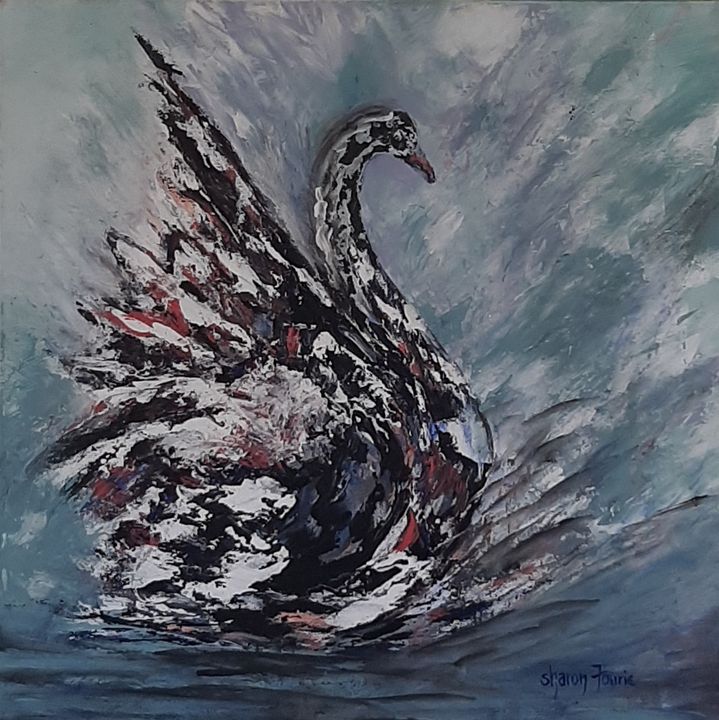This captivating abstract painting by Sharon Torrey, whose signature is displayed in the bottom right corner, features a dynamic portrayal of a swan. The swan, which occupies about half of the canvas, appears to be gracefully landing on water, creating a dramatic splash. The background is characterized by muted tones of dark gray and blue, suggesting a turbulent aquatic environment.

The swan itself is depicted with prominent, bold brushstrokes, giving it an impressionistic yet semi-realistic appearance. It primarily showcases dark black feathers with striking white, red, and blue highlights, adding depth and interest to its form. Its elongated neck, orange beak, and eye are distinctly visible, contributing to its lifelike quality. The upper left portion of the painting is marked by a notable wing, poised mid-motion, emphasizing the swan's dynamic entry into the water.

The scene is further animated by a foamy, light-colored wave that rises dramatically behind the swan, accentuating the sense of motion and splash. This visually compelling piece blends impressionistic techniques with a semi-realistic flair, making it a striking addition to any living room or office.